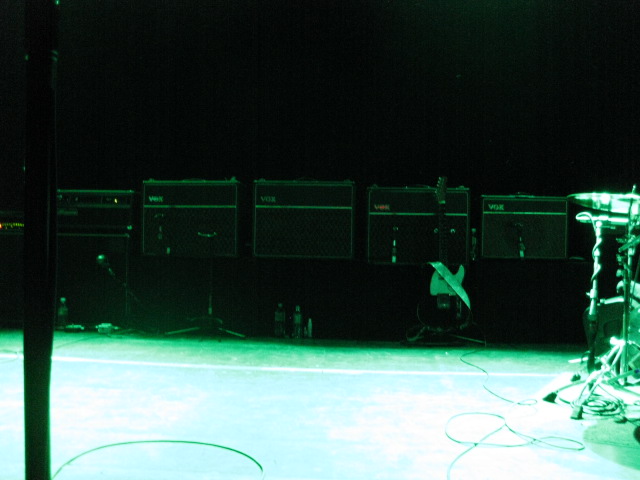The image depicts a dimly lit performance stage, accentuated by an overwhelming green tint that gives it a neon-like appearance. The background is jet black, transitioning into a gradient of green and blue hues. Along the back wall, there are several speaker or stereo boxes, some outlined or patched in green, and possibly adorned with unreadable text. At the forefront stands a guitar on a stand, positioned in front of one of these speaker boxes. Near the center, there's a bright green semi-circle and a green pole that fades to black as it reaches the top. The floor, illuminated bright green by the photograph's lighting, contrasts with the dark background. To the right-hand side, part of a drum set is visible, including a cymbal and wires extending from it back to the amps. Scattered around the stage are various wires and a few small bottles, adding to the cluttered but intimate sense of a live music setup. A microphone stand is positioned on the very left-hand side of the image.